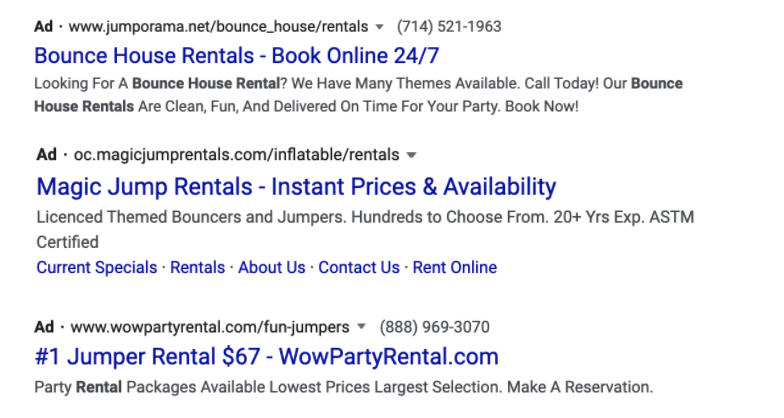This screenshot captures a segment of search results that prominently displays three sponsored ads related to rental services for inflatable bounce houses. The search platform is not identifiable as the search bar is missing, but it appears these ads emerged from a search concerning bounce house or jumping rentals.

1. The first ad, from jumparama.net, promotes their service for bounce house rentals, emphasizing the convenience of booking online 24/7.
2. The second ad, from Magic Jump Rentals, highlights their instant pricing and availability features.
3. The third ad, from Wow Party Rental, offers fun jumper rentals starting at $1.69.

Each ad features a bold "Ad" label in black typography, while the company names and links are in a darker blue color, making them stand out to potential customers seeking inflatable bounce house rentals for events or parties.